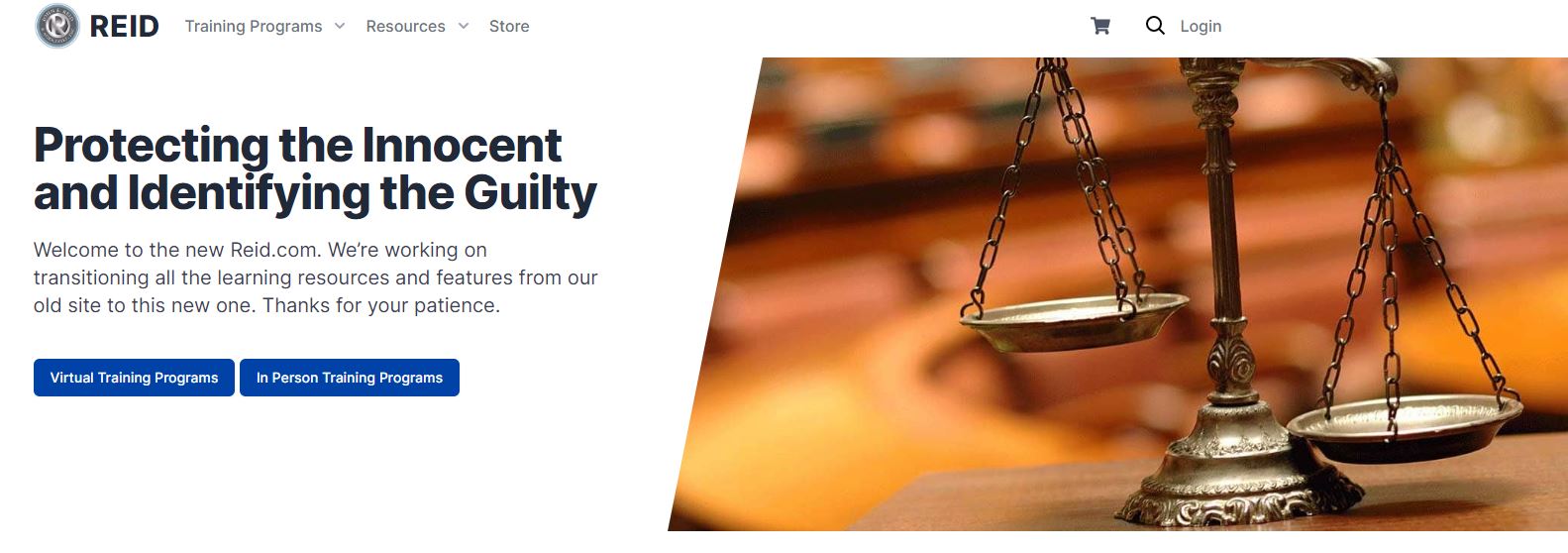This is the home page for a lawyer's office.

On the left side, the background is predominantly white. In the upper left corner, there is a circular emblem, followed by bold black text that reads "Read." To the right of this, in lighter and thinner text, there are menu options: "Training Programs" with a drop-down menu, "Resources" with a drop-down menu, and "Store."

Just below these menu options, in bold black text, is the office's mission statement: "Protecting the Innocent and Identifying the Guilty." Beneath this header, in smaller black text, a welcoming message states, "Welcome to the New Read.com. We're working on transitioning all the learning resources and features from our old site to the new one. Thanks for your patience."

Below this message, there are two blue rectangles side by side. The left rectangle contains white text that reads "Virtual Training Programs," and the right rectangle also contains white text that reads "In-Person Training Programs."

To the right of these elements, there is an image of a bronze scale of justice. The right side of the scale is lower than the left, indicating imbalance. This scale is set within a courtroom environment, depicted in the background with blurred shades of medium-rich brown.

At the top right corner of the page, there is a shopping cart icon, followed by a small black magnifying glass icon, and text that says "Log In."